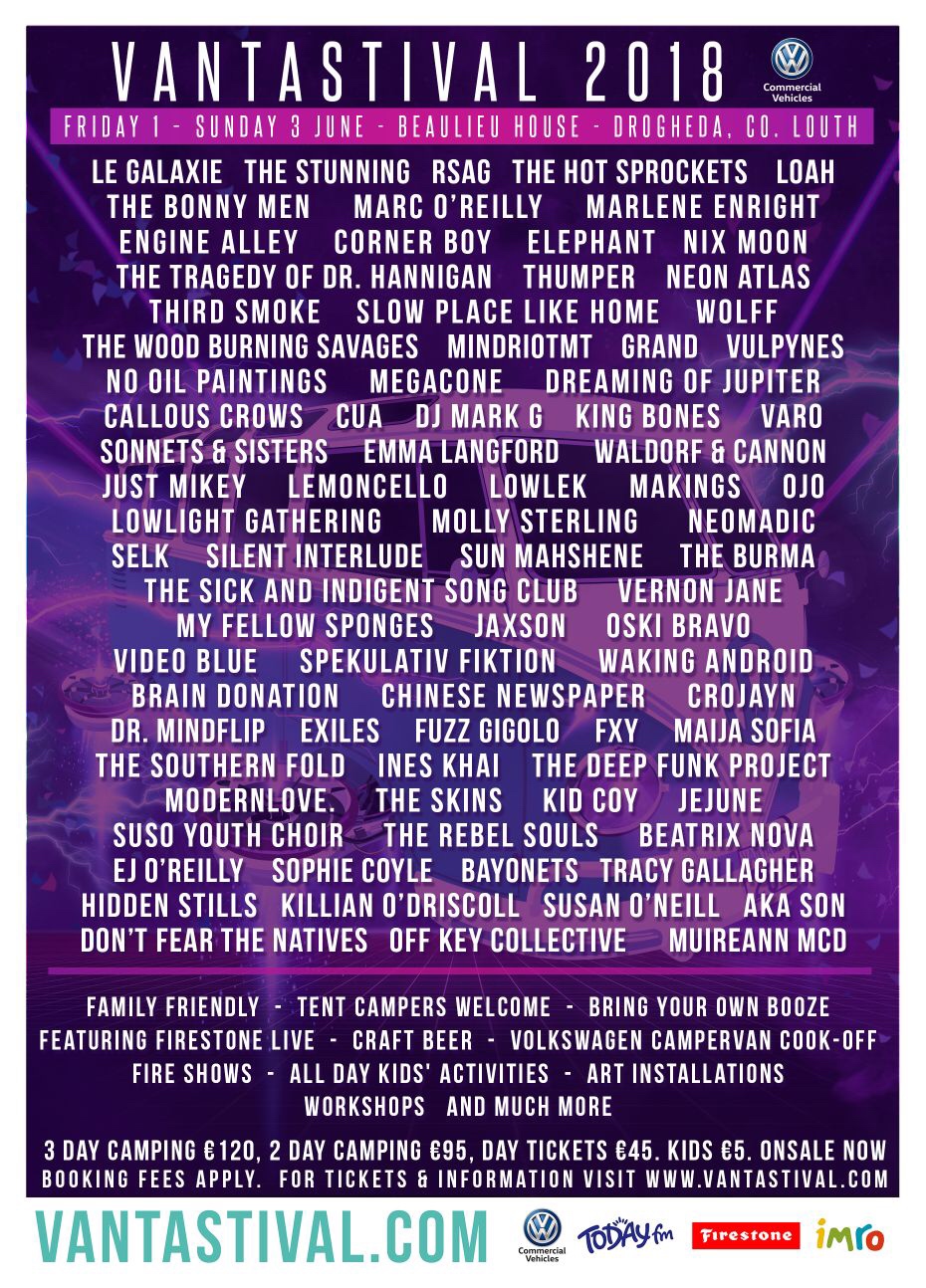This vivid and detailed promotional poster for Vantastival 2018, sponsored by Volkswagen Commercial Vehicles, is drenched in various shades of purple with intricate abstract illustrations in the background. Set to take place from Friday, June 1 through Sunday, June 3 at Bellurgan House, Drogheda, Co. Louth, Ireland, the event promises a family-friendly atmosphere with a generous list of amenities and activities. Attendees can look forward to live performances by a wide array of bands listed in predominant white text, including names like Le Galaxy, The Stunning, The Hot Sprockets, The Bonnymen, and many more. Key features of the event include Firestone Live, a Craft Beer Festival, a Volkswagen Camper Van Cook Off, fire shows, all-day kids activities, art installations, various workshops, and much more. Camping for the three-day festival is priced at 120 Euros. For further details, tickets, and more information, the poster directs viewers to visit vantastival.com, with sponsors such as Volkswagen, Firestone, Today FM, and IMRO prominently listed.